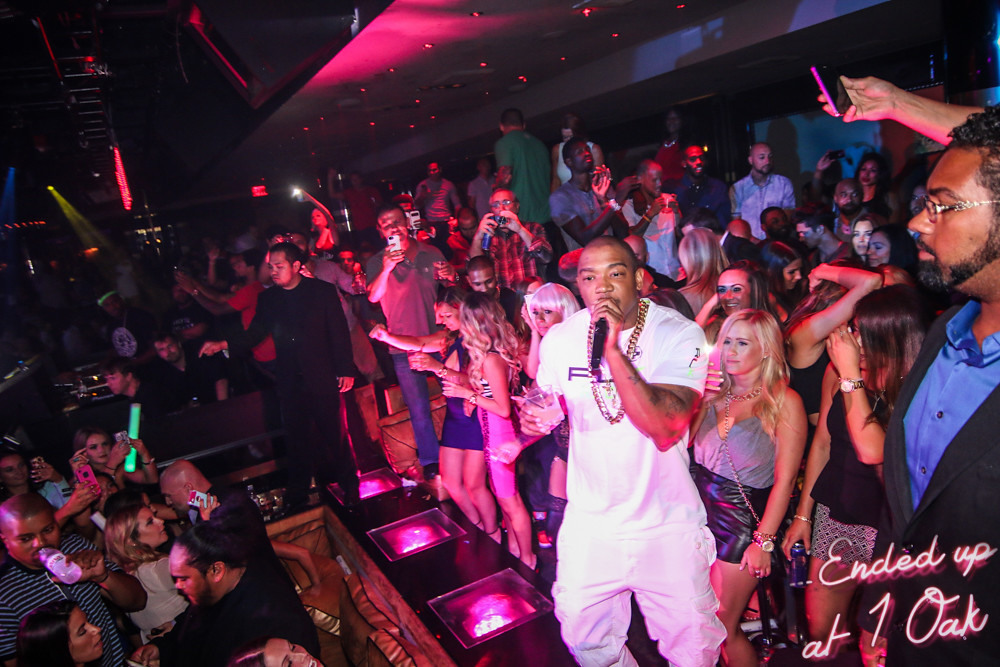In the dimly-lit interior of a nightclub, an electrifying concert is underway, as indicated by the text "Ended up at One Oak" in the bottom right corner. The room is illuminated with vibrant colored spotlights, capturing the essence of nightlife. At the center-right of the image stands a black man, identified as the rapper Ja Rule, energetically performing. He is dressed in a white short-sleeved shirt and matching white pants, accented by a large gold chain. Ja Rule holds a microphone in one hand and a drink in the other, engaging the diverse crowd around him. The background reveals a sea of people, both men and women of various ages and races, dancing and capturing the moment with their phones. To the far right edge, another man, wearing glasses, a blue dress shirt, and a black sport coat, can be seen holding up a phone over the vibrant, bustling scene. The atmosphere is one of pure enjoyment and celebration, highlighting the spirited crowd immersed in the music and ambiance of the nightclub.